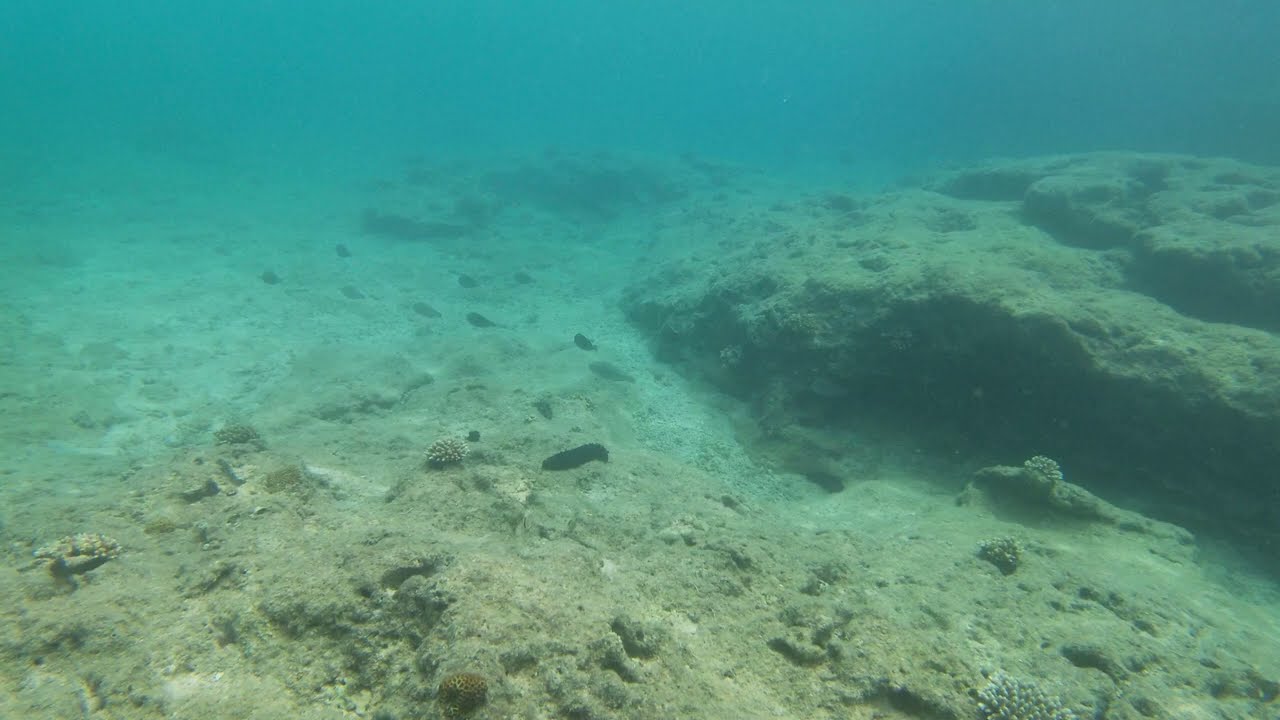This underwater photograph, presented in landscape orientation, showcases a murky aquamarine ocean scene with a notable rock-strewn seafloor. The rocky terrain, lacking in colorful coral, is covered with green moldy patches and possibly some algae or plant life, creating a muted palette of beige to dark brown variations across the ocean floor. Dominating the scene is a substantial rock outcropping that begins about a quarter of the way down from the top, extending from the right-hand side of the image towards the center. This rock formation includes a dark cavity beneath it, suggesting a potential hideaway for underwater creatures. In the middle distance, under the surface rocks, a small school of approximately a dozen slender fish can be seen swimming from left to right, blending with the natural flow and gradient of the aqua-colored water, which deepens to a darker blue as it recedes into the background. The photograph captures the realism of the underwater world, presenting an authentic representation of the ocean floor's varied textures and subdued hues.